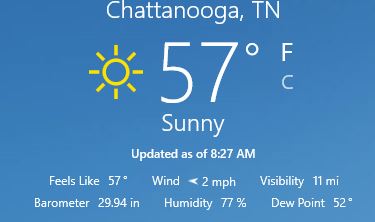Screenshot showcasing the current weather conditions in Chattanooga, TN. The background features a blue gradient, transitioning from a deep blue at the top to a lighter blue at the bottom. Centrally displayed is a bright sun icon indicating sunny weather. The temperature reads 57°F, with the 'F' in white and the 'C' in blue. 

Additional weather details include:
- Updated timestamp of 8:27 AM.
- Feels like temperature mirroring the actual at 57°F.
- Wind speed at a gentle 2 mph.
- Visibility extending to 11 miles.
- Barometric pressure recorded at 29.0 inches.
- Relative humidity at 77%.
- Dew point measuring at 52 degrees.

The screenshot encapsulates a clear, sunny morning in Chattanooga, portrayed across a visually pleasing blue gradient backdrop.